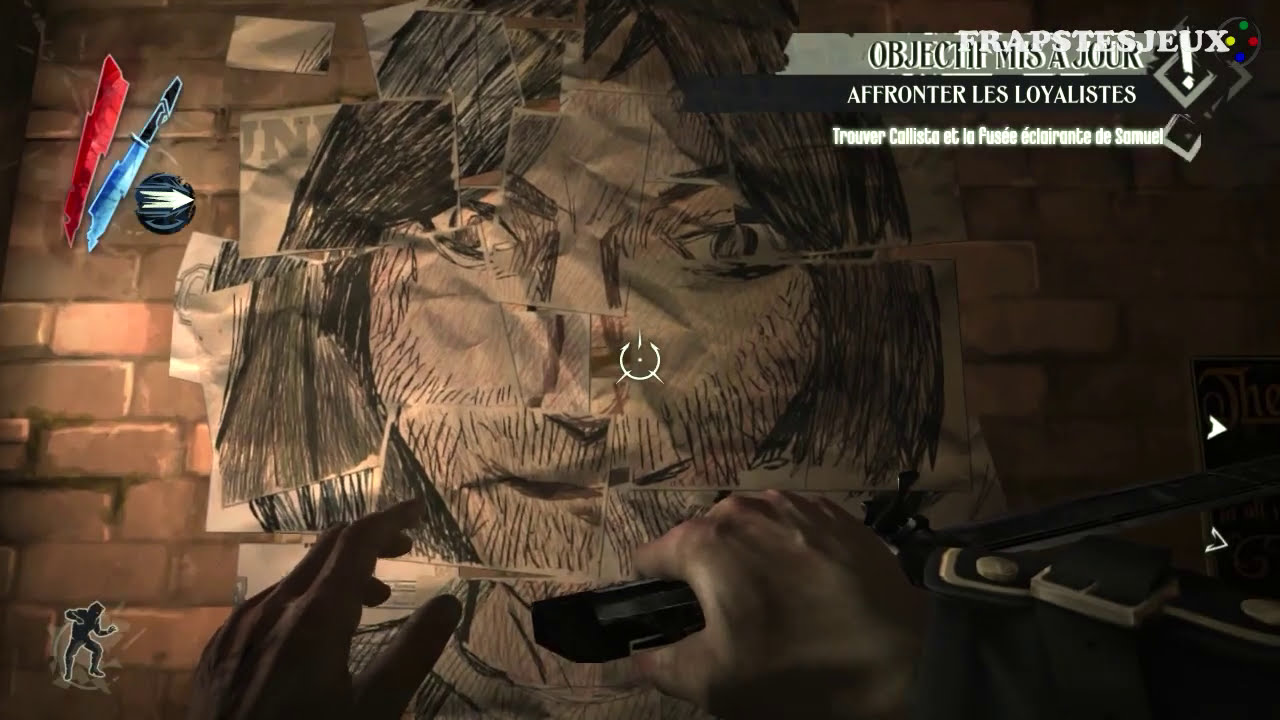The image appears to be a meticulously crafted collage of torn brown paper with intricate black pencil drawings, all reassembled and glued onto a brick wall. Central to the composition is a fragmented yet coherent depiction of a person with long black hair that nearly reaches their shoulders. The person's eyes are markedly cross-eyed, both staring outward, and their nose appears offset, further adding to the surreal nature of the artwork. Most notably, there is a bullseye located at the center of the face, and the person's mouth is partially obscured by hands; the right hand grips a black item while the left hand's fingers are open and splayed. 

In the upper left corner, two pens—one red and one blue—and a circled arrow add to the enigmatic symbolism of the piece. Below these elements, a small black caricature of a figure in a fighting stance stands out in the bottom left corner. 

On the upper right side, a block of white text begins with “Vrapshtes Jeux,” followed by “Objekts mis ajor” against a gray backdrop with white-lined letters. The text continues with “Y frontier les loyalistes” and culminates in “Trever kelista et la posse déclarante de Samuel” in glowing white letters. Below this section, three dots in green, yellow, red, and blue are arranged in a line. 

Furthermore, two arrows on the bottom right point to the right; the top arrow is solid, while the bottom one is an outline with a transparent center. The collage as a whole seems reminiscent of a medieval portrait given its stylistic elements and fragmented presentation, suggesting a blend of historical and contemporary artistic influences.